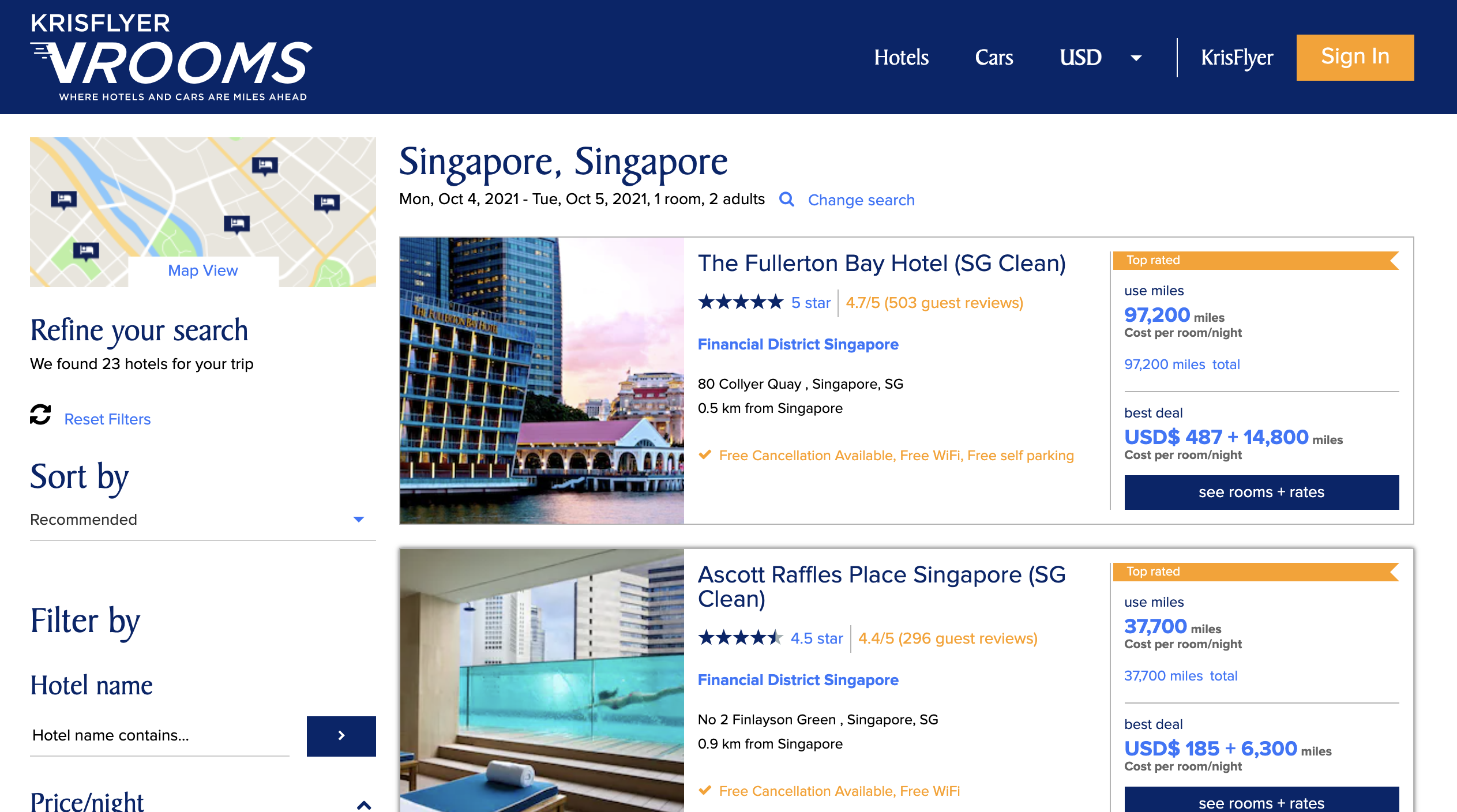Here is the improved and detailed caption:

---

A detailed screenshot of the Chris Flyer vRooms platform is displayed, showcasing the user interface for booking hotels. At the top, a blue banner with white menu text provides navigation options, while an orange sign-in button is prominently situated in the top right corner for user account access. On the upper left of the screen, there is a map view section to assist in visualizing hotel locations, directly beneath which the prompt "Refine Your Search" is positioned.

The system has successfully located 23 hotels suitable for the specified trip, searchable through various filters on the left-hand side of the screen. A "Reset Filters" button featuring circular arrows offers an easy way to clear all applied filters. 

The search parameters define a stay in Singapore, from Monday, October 4th, 2021, to Tuesday, October 5th, 2021, for one room accommodating two adults. The top search result highlights the Fullerton Bay Hotel, which boasts a five-star rating and an impressive guest score of 4.7 out of 5.